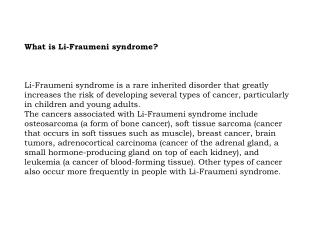This is a low-resolution screenshot of a text-only document or webpage with a plain white background and black text. The top of the image features bold text that reads, "What is Li-Fraumeni Syndrome?" The body of the text explains that Li-Fraumeni Syndrome is a rare inherited disorder that significantly increases the risk of developing various types of cancer, particularly in children and young adults. The cancers associated with Li-Fraumeni Syndrome mentioned in the text include osteosarcoma (a type of bone cancer), soft tissue sarcoma (a cancer occurring in soft tissues such as muscle), breast cancer, brain tumors, adrenocortical carcinoma (a cancer of the adrenal gland, which is a small hormone-producing gland located on top of each kidney), and leukemia (a cancer of blood-forming tissues). The text also notes that other types of cancer occur more frequently in individuals with this syndrome. Given the specific medical terminology and detailed explanations, the screenshot likely originates from a medical document or a peer-reviewed research study, although it could also be from an authoritative medical information website. The precise source, however, remains unclear from the image alone.